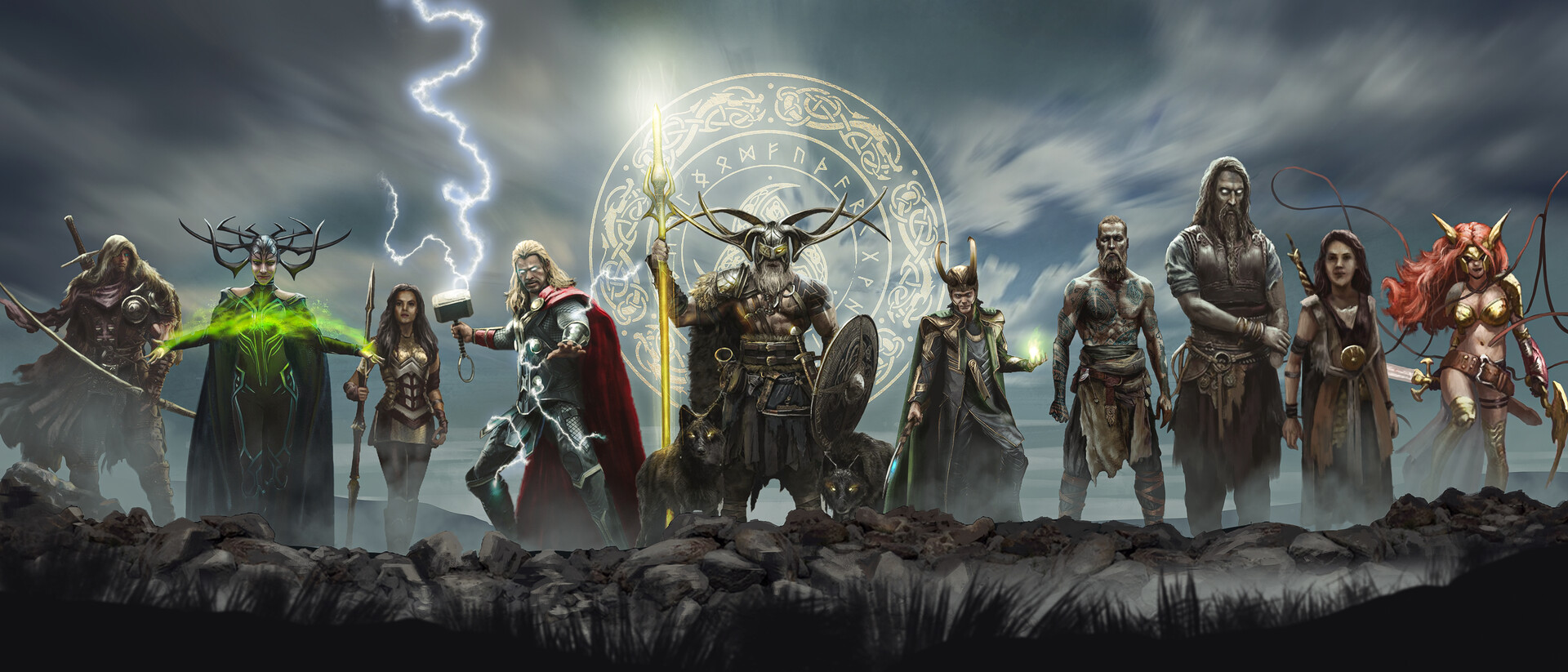The artwork showcases ten Marvel characters, prominently featuring Thor amidst a dark and stormy, cloud-filled background. Thor, wielding his hammer with lightning extending from it to the sky, stands fourth from the left. The characters are arranged standing on a rocky area with sparse grass beneath their feet. Behind them, a circle adorned with runes or mystical writing adds to the dramatic atmosphere. On the far left is a man brandishing a large sword. Next to him, a woman emits green energy from her outstretched arms, accented by helmet-like tree branches. A blonde woman holding an impressive spear stands near Thor. Central to the scene is a muscular man grasping a staff with horns, flanked by two wolves. To his right is an ominous figure, possibly Loki, holding a weapon in one hand and a green orb in the other. The remaining characters, inspired by Norse mythology, include a man with a horned helmet and a final fierce-looking woman with flaming red hair and a gigantic whip and sword, all poised as though ready for battle.